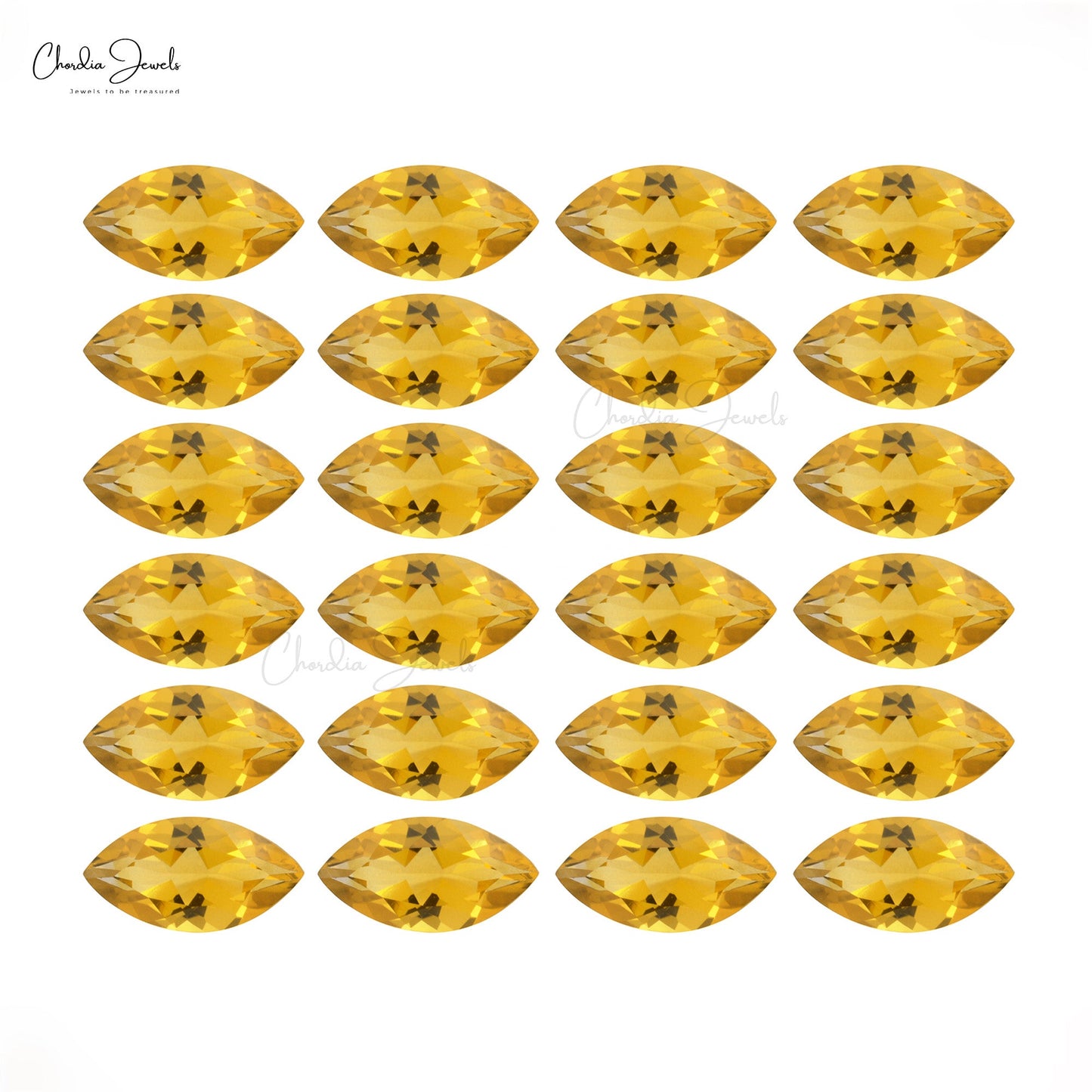The image depicts a web advertisement or webpage for Chandia Jewels, featuring a clean all-white background adorned with football-shaped gemstones arranged symmetrically. The top left corner of the image displays "Chandia Jewels" written in elegant cursive, along with the tagline "Jewels to be treasured." A faint "Chandia Jewels" watermark appears twice in the center portion of the image, each in a light gray hue. The gemstones are organized into six rows and four columns, totaling 24 oval-shaped jewels. Each gemstone features a golden, apple-juice color with intricate striations and varying shades of gold, some with tiny black smudges. These gemstones, which possess a crystallized look, are spaced evenly apart, both vertically and horizontally, adding to the symmetrical and geometrical aesthetic of the artwork.